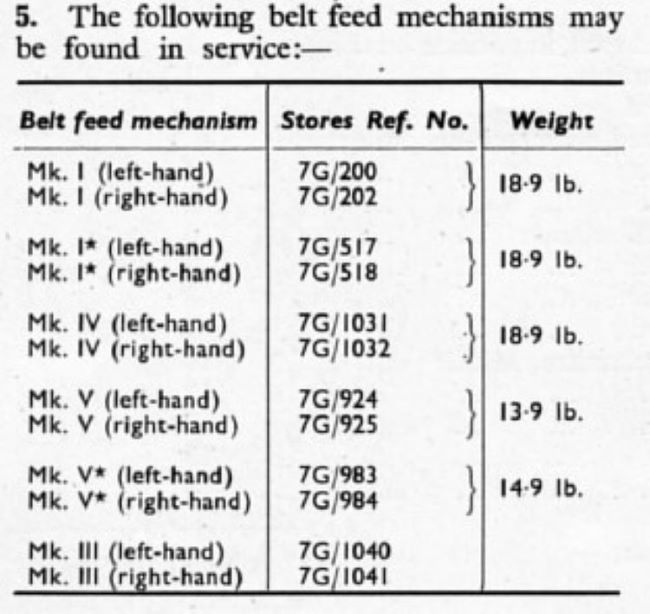The image displays a scanned or photographed document against a white background, featuring black text. At the top, it reads "5. The following belt feed mechanisms may be found in service," followed by a dash, leading into a detailed three-column chart. The first column is titled "Belt Feed Mechanism" and lists various mechanisms, including "Mk1 (Left Hand)," "Mk1 (Right Hand)," "Mk1* (Left Hand)," "Mk1* (Right Hand)," "Mk4," "Mk5," "Mk5*," and "Mk3," all in the same left-hand and right-hand format where applicable. The second column, titled "Stores Ref No.," aligns specific reference numbers with each belt feed mechanism: 7G/200, 7G/202, 7G/517, 7G/518, 7G/1031, 7G/1032, 7G/924, 7G/925, 7G/983, 7G/984, 7G/1040, and 7G/1041. The third column, titled "Weight," lists corresponding weights: 18.9 pounds for Mk1 and Mk1*, 13.9 pounds for Mk4, 14.9 pounds for Mk5*, and weights listed accordingly for other mechanisms.